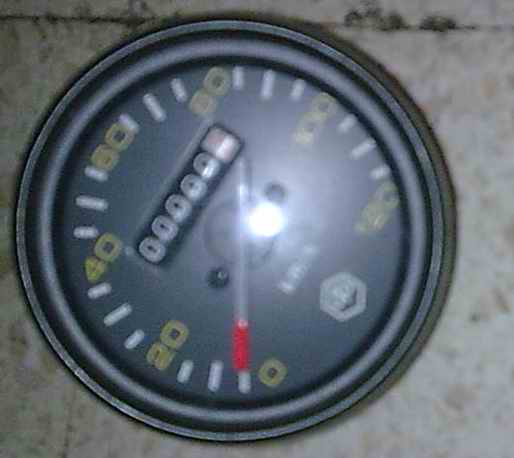In this blurred image, a circular odometer, possibly from a motorcycle or moped, is prominently displayed. The odometer features a black outer casing with a glossy glass cover. A white needle with a red tip sits at the center, poised to track speed variations as the vehicle moves. The speedometer's scale, marked in yellow and white, displays incremental numbers: 0, 20, 40, 60, 80, 100, and 120, with smaller white tick marks in between each numeral. At the center of the dial, a mechanical odometer shows a mileage reading of all zeros. Although the image is too fuzzy to discern fine details, a logo with a four-sided, almost hexagonal shape is visible at the bottom. Above this logo is some illegible writing, accompanied by a circle featuring two black dots. A light reflection on the glass cover further obfuscates the details, adding to the image's overall lack of focus.